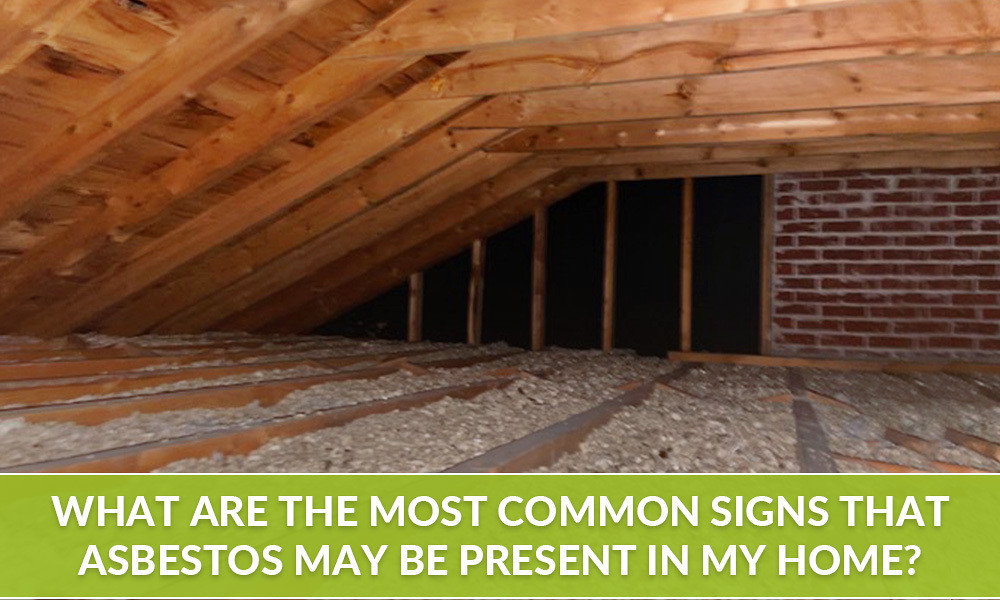This image depicts a dimly lit attic with unfinished wood beams forming the low roof structure and visible brick panels in the background. The floor is layered with wooden beams and what appears to be insulation material. On the left side of the image, a dark area framed by thin wooden beams contrasts against the brick wall to the right. At the bottom of the photo, a green rectangular box with white text poses the question: "What are the most common signs that asbestos may be present in my home?" suggesting an informative advertisement about asbestos detection.